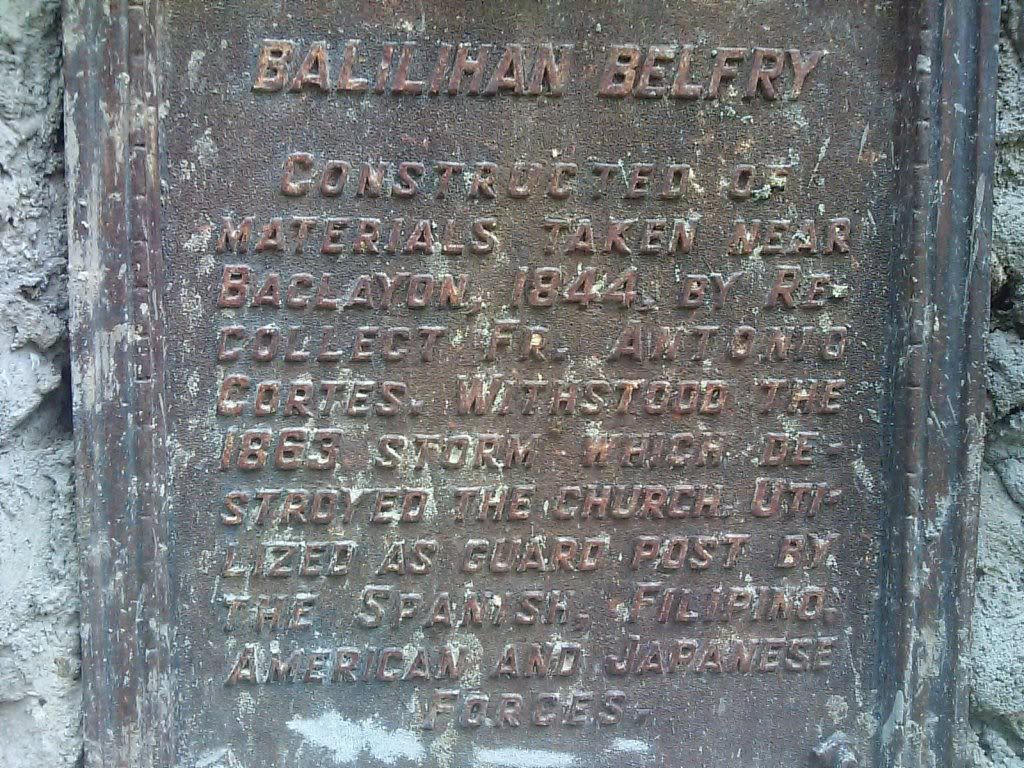The image depicts an aged copper plaque mounted on what seems to be a stone or cement wall. The plaque, which has developed a brownish patina over time, features raised capital letters. Although partially obscured by a watermark that includes a circular logo and the words "photo bucket" with "protect more of your memories for less," some text is still readable. It prominently states "Balilijan Belfry constructed of materials taken near..." with the year "1884" visible. Further down, it mentions, "withstood the 1863 storm which American and Japanese forces," indicating its historical significance related to events that may involve World War II. The plaque itself appears to be weathered with some white chips, adding to its vintage character.